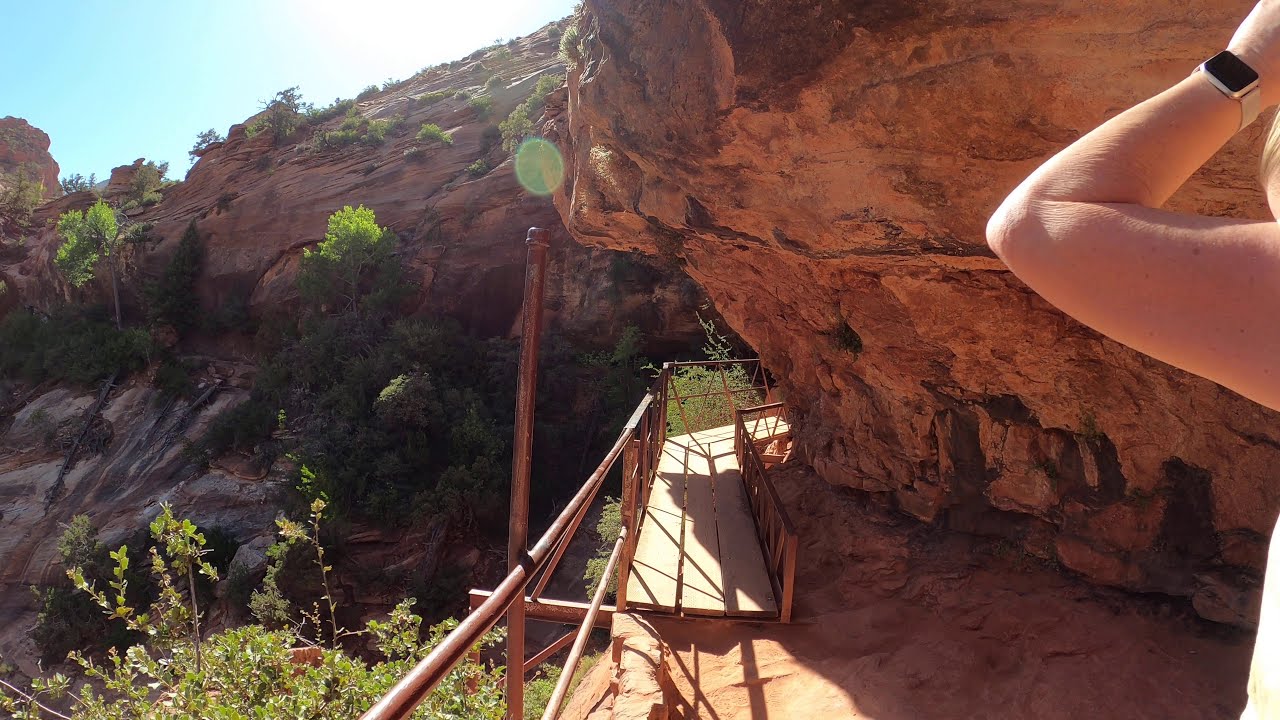This detailed photograph captures a scenic outdoor setting, likely within a national park or near the Grand Canyon. Dominating the center of the image is a smooth, light brown walkway with metal railings on either side, designed to guide visitors across a rugged terrain. This bridge-like structure, a dark tan color matching the surrounding dirt, angles to the right around a prominent rock formation that arches over part of the path. 

To the right of the image, there is a woman's arm raised, adorned with what seems to be an Apple Watch, recognizable by its black interface and light-colored band. The arm, appearing to be of a Caucasian individual, is partially veiled against a backdrop of rusty and orangish-brown rocky cliffs that rise steeply on both sides, suggesting the path traverses a narrow canyon or underpass.

The rock formations, towering high into the sky, exhibit varying shades of brown, interspersed with patches of green from trees and bushes. At the top left of the photograph, a serene light blue sky is visible, indicating a sunny day. This picturesque scene, devoid of any text, vividly illustrates the natural beauty and rugged charm of the outdoors, providing a glimpse into an adventurous trailside experience.